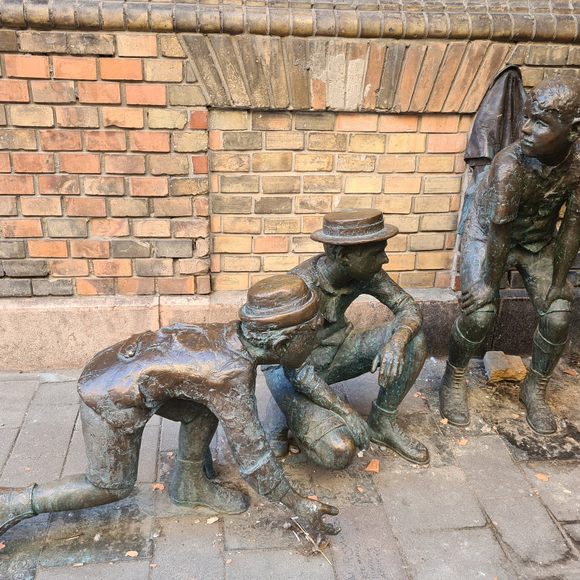The photograph captures an outdoor scene featuring a metal, likely bronze, statue of three young boys in vintage costumes arranged in front of a varied pink, red, and yellow brick wall. The statues are set on a cement brick paver sidewalk. The first boy on the left is kneeling on one knee, bent down with his hand on the ground, as though he is rolling dice, and he wears a small hat. The middle boy is also kneeling, resting his left arm on his knee, watching the ground intently while wearing a flatter-rimmed hat. The boy on the right is crouching higher than the others, with his hands on his knees, looking off to the left side of the photograph. All the boys are depicted in a bronzish-greenish patina color and wear short boots, creating a vintage and cohesive scene that gives the impression of play or a game in progress.